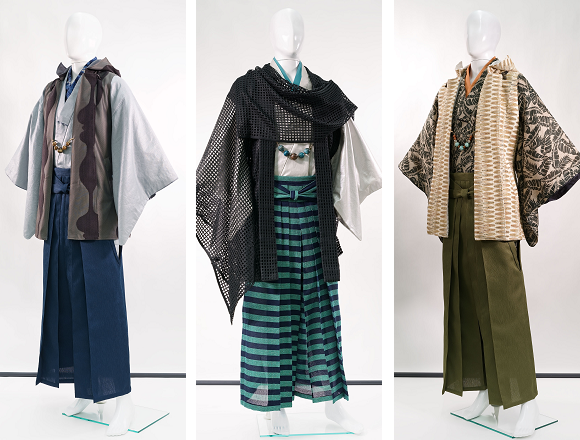The image is composed of three separate tall rectangular photos placed side-by-side, each depicting a white mannequin wearing a different detailed outfit. The mannequins are positioned against a plain background, emphasizing the clothing.

Starting from the left, the mannequin features wide-leg dark blue pants paired with a gray cape that has a fur lining. Over this, a long vest with wide sleeves adds depth to the ensemble.

In the center, the mannequin sports dark green plaid wide-leg pants and a loose-fitting white blouse. Draped over the blouse is a black cape, and the outfit is accessorized with a unique greenish and brown turquoise necklace, adding a touch of elegance.

On the right, the mannequin is dressed in green wide-leg pants and a green cape top. Over this, a patterned brown sweater with leaf-like black prints creates a textured look.

Each mannequin faces a different direction, creating a dynamic display of the clothing against the clean, unobtrusive background, highlighting the textures, patterns, and layers of each outfit.